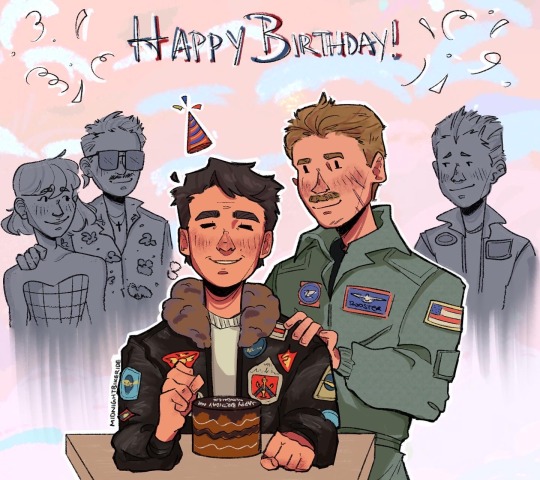The image shows a detailed 'Happy Birthday' card with a pinkish background and "Happy Birthday" written in a grayish-white text with a gray border. Intricate party designs, including circular patterns and triangles, adorn the top left and upper right corners. Dominating the foreground is a man in a brown bomber jacket with a collar and patches, reminiscent of military attire, suggesting a theme from the movie "Top Gun." He is seated in front of a two-layered chocolate cake. His left hand rests on the table, while his right hand is raised in a celebratory fist above the cake. 

To his right, another man in an all-green army outfit, featuring an American flag patch on his left shoulder and additional patches, stands proudly with his arm draped over the birthday celebrant’s shoulder. This character is identified as "Rooster," marked by his mustache and parted hair. In the background, three people are attentively looking forward, and cloud patterns in pink and sky blue add a dreamy effect to the scene. A celebratory mood is evident, enhanced by a sense of camaraderie and homage to "Top Gun."